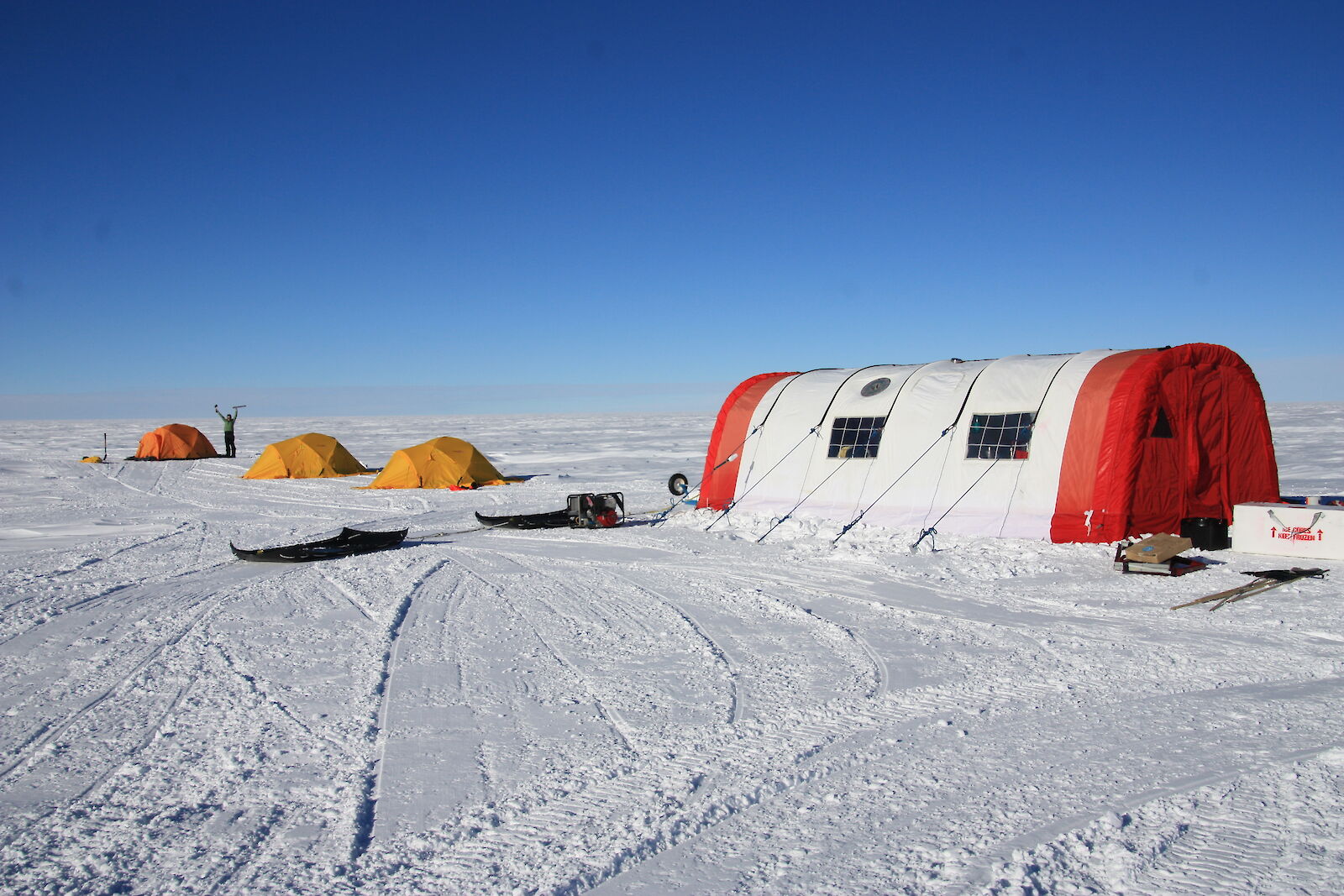In this horizontally aligned rectangular picture, taken in a cold climate, the top part showcases a stunning, solid clear blue sky. From the middle down, the landscape transitions into a vast, flat expanse covered entirely in snow, punctuated by numerous tire and snowmobile tracks. Prominently featured is a large, arch-shaped tent located on the middle right side just below the sky. This tent, likely serving as a research or common area, has distinctive red dome-shaped ends and an extended white arched section in between. It is anchored securely to the ground with four or five tightly drawn ropes. The tent’s sides feature two black windows with white lines forming small squares, adding to its utilitarian design. 

In the foreground, tracks from various vehicles crisscross the snow-covered land, possibly marking frequent routes of travel. Off in the distance, toward the middle left, three smaller, dome-like tents dot the landscape—two are yellow, and one is orange. Near the orange tent, a person stands with their hands raised, possibly holding something. There are also some ski boards or surfboards on the ice nearby. Alongside the large tent, some boxes and equipment are visible, including one box marked "keep frozen." The entire scene is illuminated by bright sunlight, reflecting off the pristine snowy surface, painting a picturesque and lively snapshot of an arctic-like outdoor expedition.